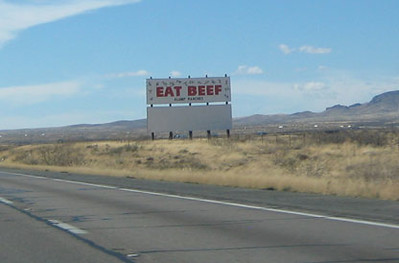A roadside billboard, captured from the passenger side window of a car, prominently displays the message "EAT BEEF" in large, bold, red letters against a white background. Directly beneath it is a blank billboard, awaiting its future message. Both billboards are supported by five tall wooden poles arranged from left to right. The surrounding landscape is flat and arid, with patches of dry, dead grass interspersed with small spots of green, characteristic of a desert-like environment. In the distance, brown dirt gives way to the peaks of mountains or very large hills, adding depth to the scenery. The image also includes a two-lane road running parallel to the billboards. Above, the sky is a light blue, adorned with a few wispy, light clouds, completing the picturesque view.